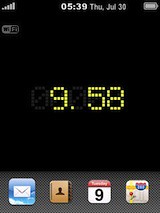The image is a detailed screenshot of an iPod or iPhone interface with a black background. At the top-left corner, there is a Wi-Fi symbol displaying five bars, with the word "Wi-Fi" underneath it. Next to it, the time reads "05:39" and the date is "Thursday, July 30th." On the top-right corner, there is a fully charged battery symbol. 

In the center of the screen, the time "9:58" is prominently displayed. At the bottom of the screen, there is a gray banner with four distinct icons arranged in squares. The first square on the bottom left has a background of a blue sky with a white envelope, indicating an Email application. The second square, also on the bottom left, features a tan background with a black silhouette of a head, representing Contacts. The third square on the bottom right displays a white calendar with the numerical date "9" and a red top, signifying a Calendar app. Finally, the fourth square on the bottom right shows a map icon with yellow roadways and an interstate sign, representing a Maps application.